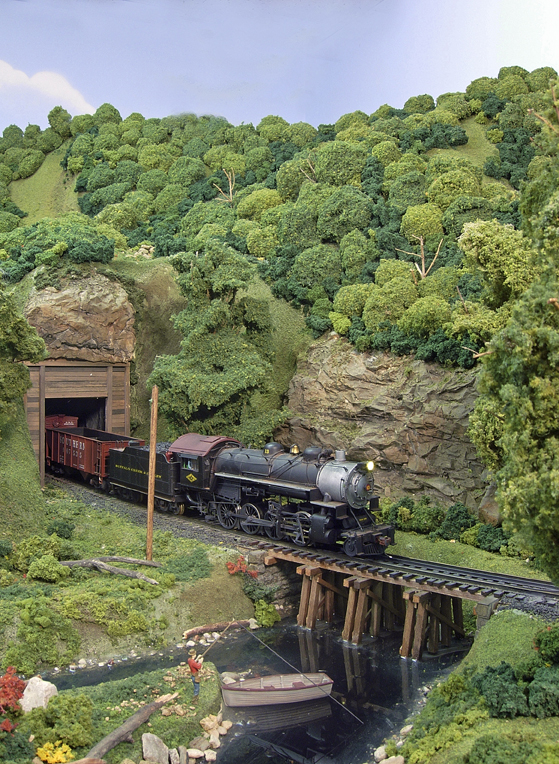In this image, a vintage freight train is emerging from a brown tunnel nestled within a lush, green forest landscape. The front of the train is black, followed by cars with a mix of reddish roofs and black sections, suggesting an older era. The train navigates a bridge supported by three pillars that span a serene stream or lake below. The sky is primarily blue adorned with fluffy white clouds. On the grassy riverbank in the foreground, a man dressed in a red shirt, blue pants, and a hat is fishing beside a small rowboat. The detailed scenery includes green trees, shrubbery, brown rocks, and flowers, adding to the picturesque setting.